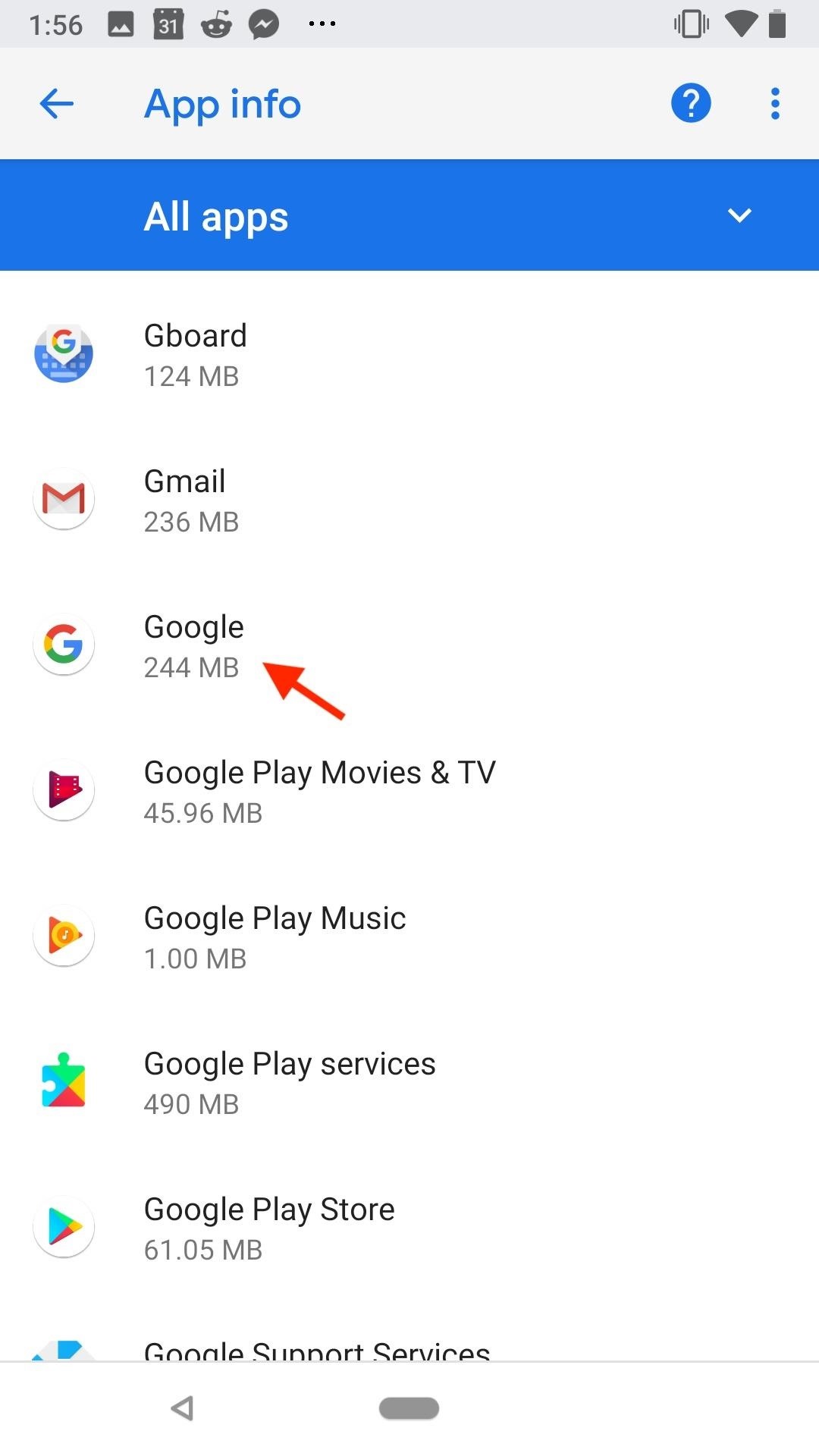This screenshot, captured from a cell phone, displays the "App Info" tab under the Settings menu. The interface adopts a clean and minimalist design with a predominant white background.

At the very top of the screen is a dark gray status bar. On the left side, the current time is visible. Adjacent to the time are five icons, though their specific details are not mentioned. On the right side of this bar, the status details display the signal strength, Wi-Fi connectivity, and battery level.

Below the status bar is a pale gray navigation bar. Prominently placed on the left are the words "App Info" highlighted in blue, next to a blue left-facing arrow. On the right side of this bar, there is a blue circle with a white question mark inside it, likely for a help option, followed by a vertical ellipsis (three vertically aligned dots), indicating that additional options are available through a menu.

Underneath this navigation bar is a blue tab containing a white text label "All apps" on the left and a white drop-down arrow on the right side. This tab serves as a filter for the list of apps displayed below.

The main content area lists various apps along with their respective icons, names, and storage usages:
1. "Gboard" is represented by a Google logo with a blue and white background and uses 125 megabytes.
2. "Gmail" follows with its recognizable logo, consuming 236 megabytes.
3. "Google" is marked by its circular 'G' logo and uses 244 megabytes. A red arrow, added by someone, points bottom-right to top-left aiming at this app's entry.
4. "Google Play Movies & TV", identified by its logo, uses 45.96 megabytes.
5. "Google Play Music" is shown with its icon and utilizes only 1 megabyte.
6. "Google Play Services" features a puzzle piece logo and occupies 490 megabytes.
7. "Google Play Store", with the Play Store logo, takes up 61.5 megabytes.
8. "Google Support Services" appears partially visible at the bottom of the list, with its full details mostly cut off from view.

Finally, at the bottom of the screen, there's a clear navigation bar integral to the phone interface, featuring a left-pointing triangle on the left-hand side, indicating a back or return function.